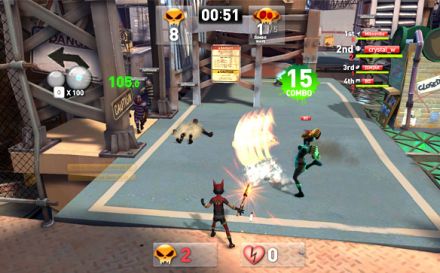In this dynamic screenshot from a video game, the central character stands with their back to the camera, brandishing a formidable weapon that radiates a vivid orange glow. Evident from the aftermath of the glowing weapon's might, several adversaries lie defeated around them. The game interface displays a time of 51 seconds at the top of the screen, indicating the duration of the ongoing action. Additional icons enrich the scene: a skull with a red "2" signifies the number of enemies vanquished, while a heart with a white "0" likely denotes remaining health points or lives. The characters engage in battle on a large blue rug bordered in white, which rests upon a sleek metal surface, adding a stark contrast between the soft textures and the industrial backdrop.